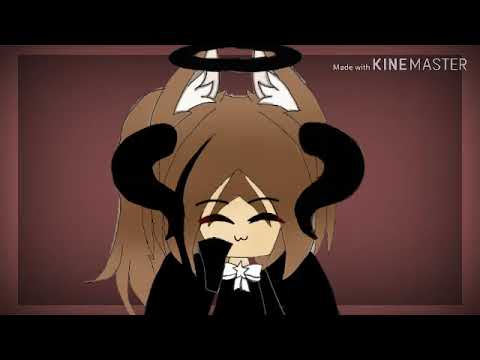The image is a screenshot from an animated video, likely an anime cartoon, featuring a single character prominently in the center. The character, who appears to be a girl, is facing forward with her head slightly bowed and smiling subtly. She has thick, brown hair with a distinctive black streak running through it and two black horns extending from the top of her head. The horns curl down the sides of her face, then turn outward at the tips. Hovering above her head is a black halo.

Her attire consists of a black robe or gown paired with a white bow tie that has a star in its center. She also has black eyebrows and horizontal strip-like eyes. There is a suggestion of tan ears with white insides peeking through her hair, likely adorned with a tuft of white fur. 

The background is largely composed of a dark red rectangle with a lighter red gradient border surrounding it, adding a sense of depth. The ground or surface at the bottom of the image is black. Additionally, there is a watermark in the top right corner of the image that reads "Made with KineMaster," indicating the screenshot originated from a video edited using this software. The overall scene is framed with black horizontal borders at the top and bottom, emphasizing it as a video capture.